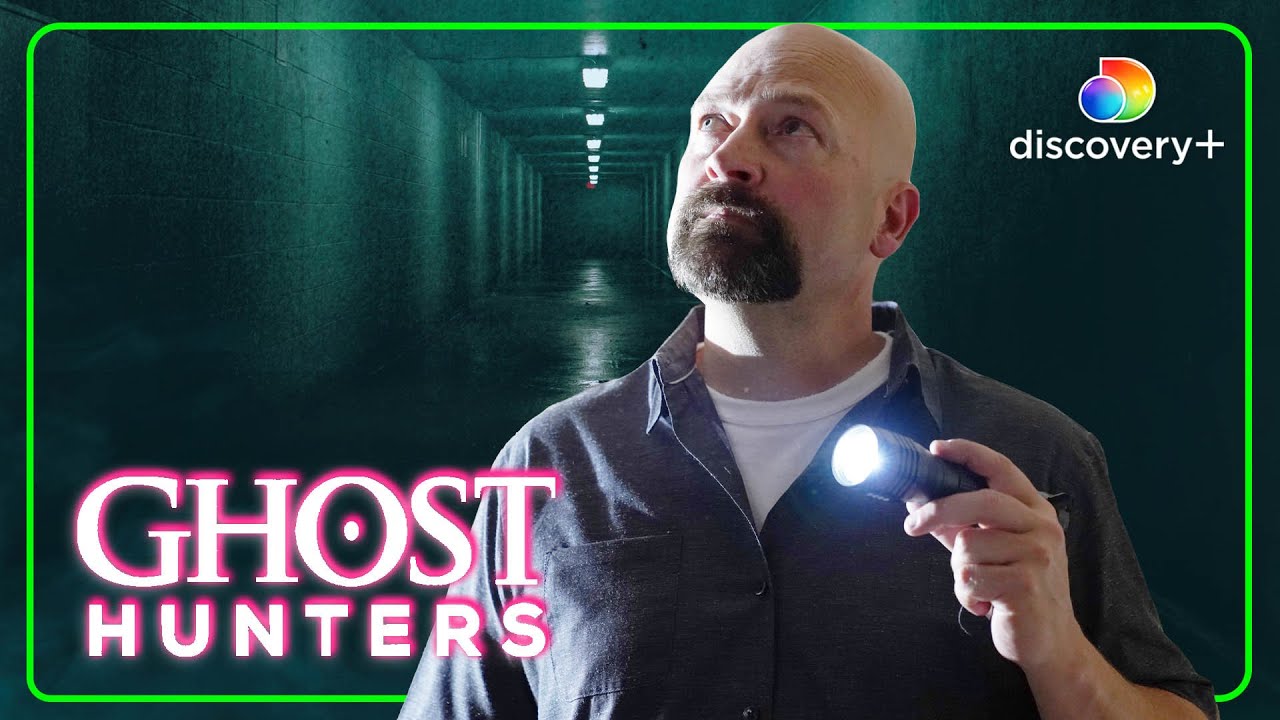The image is a promotional screenshot for the show "Ghost Hunters." It features a rectangular frame with a thin neon green border. The setting is a long, dark hallway with cinderblock walls, illuminated dimly by fluorescent lighting on the ceiling, suggesting an institutional building like a prison or asylum. In the foreground, a middle-aged, bald, white male with a dark brown goatee is seen. He is wearing a gray short-sleeved button-down shirt with the collar open and a white undershirt underneath. Holding a flashlight in his left hand, he points it upwards to his right while also looking in the same direction. The Ghost Hunters show title is prominently displayed in the lower left corner in bold, blocky white text outlined in neon pink. The upper right corner features the Discovery Plus logo, accompanied by the text "Discovery Plus."